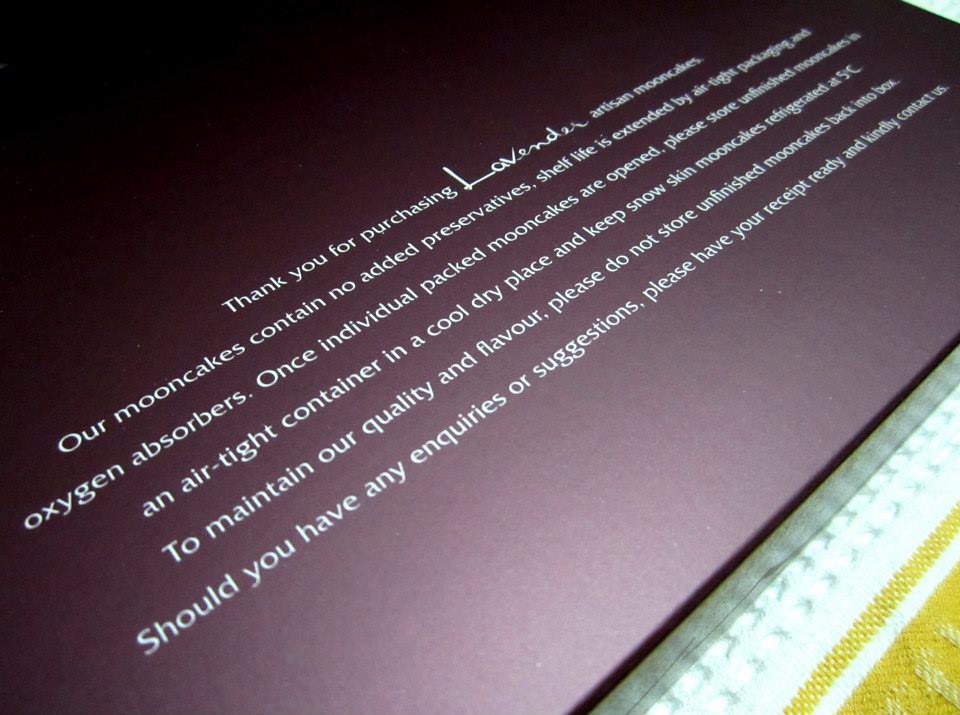This detailed photographic image captures a tilted screenshot of a thank you note, presumably part of the packaging for Lavender Artisan Mooncakes. The note is set against a predominantly purple background that starts very dark, almost black, in the upper left corner, gradually transitioning to a purple hue as it moves downward. The text is in white, slightly askew, running diagonally from the lower left to the upper right. It states, "Thank you for purchasing Lavender Artisan Mooncakes. Our mooncakes contain no added preservatives. Shelf life is extended by airtight packaging and oxygen absorbers. Once individually packaged mooncakes are opened, please store unfinished mooncakes in an airtight container in a cool, dry place, and keep snow skin mooncakes refrigerated at 5 degrees Celsius to maintain our quality and flavor. Please do not store unfinished mooncakes back into the box. Should you have any inquiries or suggestions, please have your receipt ready and kindly contact us."

In the lower right corner of the image, there is a gold-colored triangle, accompanied by a piece of fiber and a gold stitch running along the triangle’s edge, embedded in a piece of white fabric. The configuration suggests this could be a tablecloth or part of the mooncake packaging design. The primary colors in the image include varying shades of purple, maroon, white, and gold, giving it an artisanal, high-quality appearance.